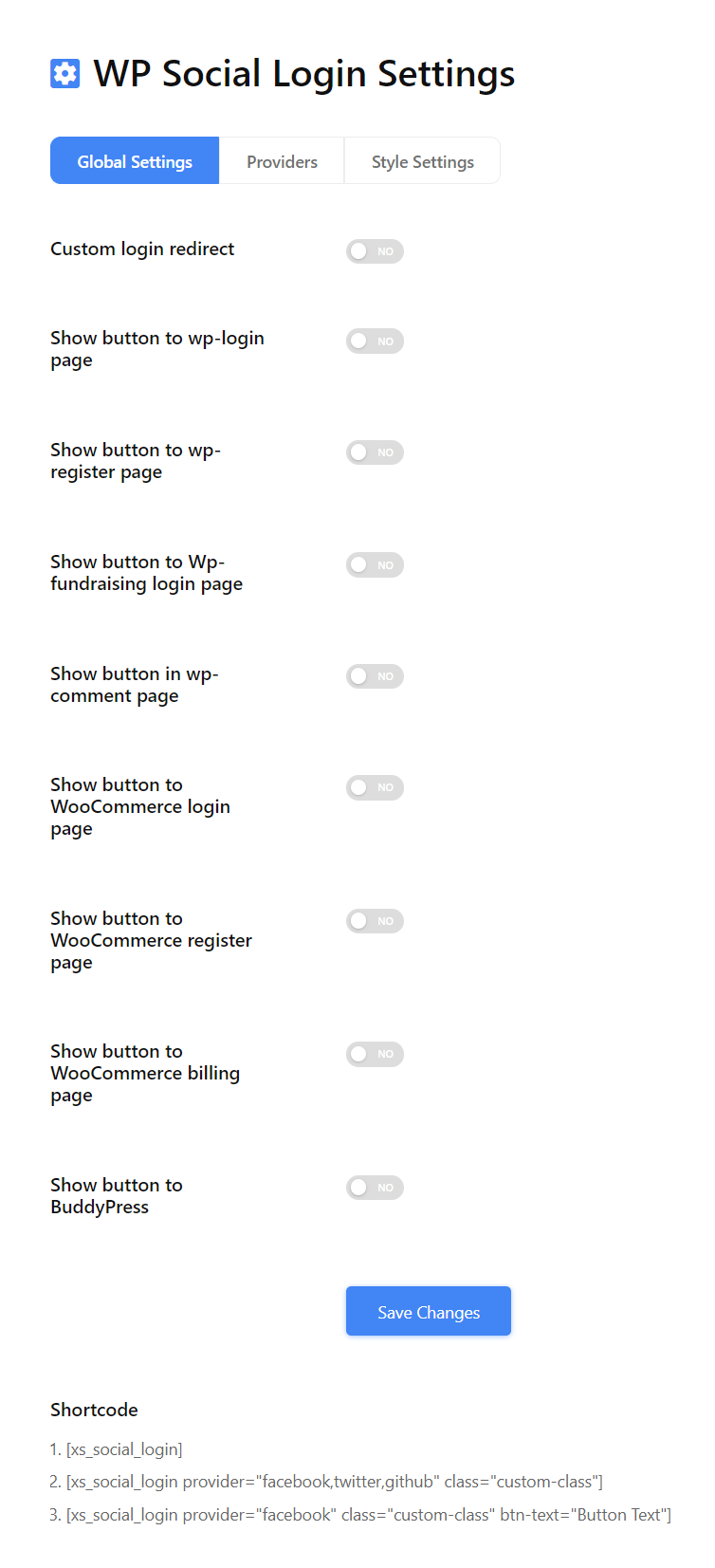Here's a cleaned-up and detailed caption:

---

This image showcases the "WP Social Login Settings" webpage with a dark-themed user interface. At the top, the title "WP Social Login Settings" is displayed prominently. Below the title, there are three horizontal tabs named "Global Settings," "Providers," and "Style Settings." The "Global Settings" tab is currently active, highlighted in blue.

In the "Global Settings" section, there is a series of options with descriptions followed by toggle switches for enabling or disabling specific settings. Each option currently has its toggle set to "No," indicated by the switches being grayed out and slid to the left. The options listed are as follows:

1. Custom Login Redirect
2. Show Button to WP Login Page
3. Show Button to WP Register Page
4. Show Button to WP Fundraising Login
5. Show Button to WP Comment Page
6. Show Button to WooCommerce Login Page
7. Show Button to WooCommerce Register Page
8. Show Button to WooCommerce Billing
9. Show Button to BuddyPress

At the bottom of these options is a blue "Save Changes" button. Below this, on the left side, there's a bolded shortcode. Adjacent to the shortcode are three different scripts, likely for users familiar with scripting and customization.

Additionally, a small gear emoji inside a blue box appears on the interface, symbolizing the settings icon.

---